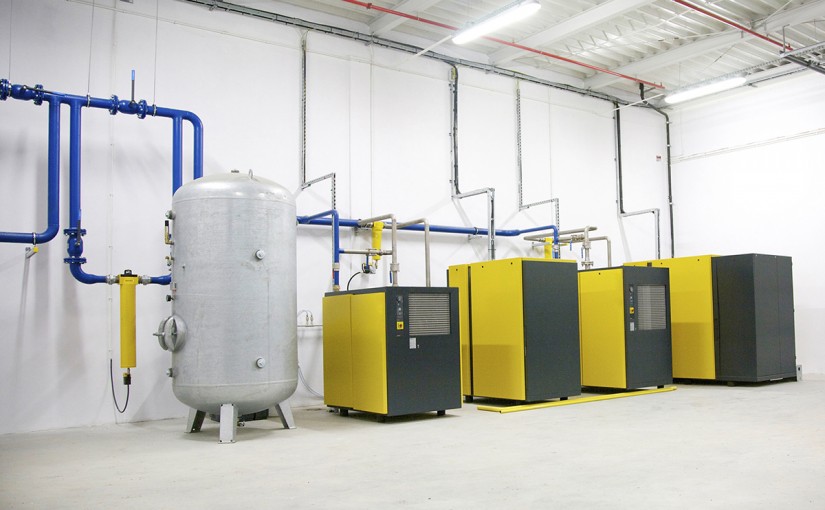The image shows the interior of a large industrial facility, possibly a factory or machinery plant, with an organized and modern appearance. The area is well-lit by fluorescent lighting mounted on the high metal roof, and the walls are painted white with no windows visible. The floor appears to be made of concrete.

Prominently featured in the foreground is a silver cylindrical object, likely a furnace or boiler, standing on four short white legs. Beyond this, a series of interconnected blue pipes with various yellow objects attached run both vertically and horizontally against the white wall. These pipes appear to connect to multiple modern machines positioned in a row from left to right.

There are five noticeable machines, predominantly in black and yellow. Each of these machines features control panels, some with front grids and various buttons. The first of these is a sleek black and yellow machine, which appears to be brand new and possibly part of an energy production system or another industrial process. Following this, there are three more black and yellow machines, each with unique configurations but similar in their modern design and functionality. The final machine on the far right is the largest among them, distinguished by its considerable size and complex interface.

The overall setup, including the pipes running along the back wall and the various machinery, conveys a highly organized industrial environment designed for efficiency and modern functionality.